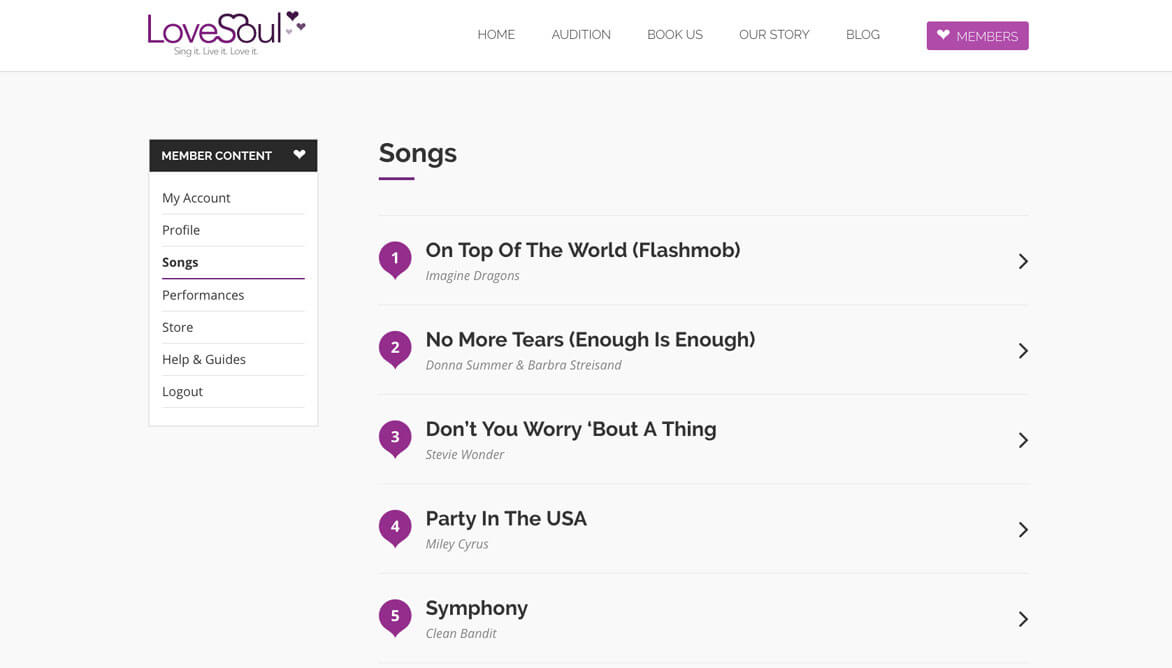The image features a website interface with multiple navigation elements. At the very top, on the left side, there is a menu item labeled "Love Soul." Centrally located at the top of the page, there are additional menu items: "Home," "Audition," "Book Us," "Our Story," and "Blog." 

To the right, there's a prominent purple box labeled "Members." Below this box, on the left sidebar, there are various options listed: "Member Content," "My Account," "Profile," "Songs," "Performances," "Store," "Helping Guides," and "Logout."

On the right sidebar, there's a section dedicated to songs. At the very top of this section, the word "Song" is displayed, followed by a thin line. Below this, there’s a lighter-colored line and a numbered list presented inside a purple text box. 

The song list includes:
1. "On Top of the World" by Imagine Dragons
2. "No More Tears (Enough Is Enough)" by Donna Summer and Barbra Streisand
3. "Don't You Worry 'bout a Thing" by Stevie Wonder
4. "Party in the USA" by Miley Cyrus
5. "Symphony" by Clean Bandit.